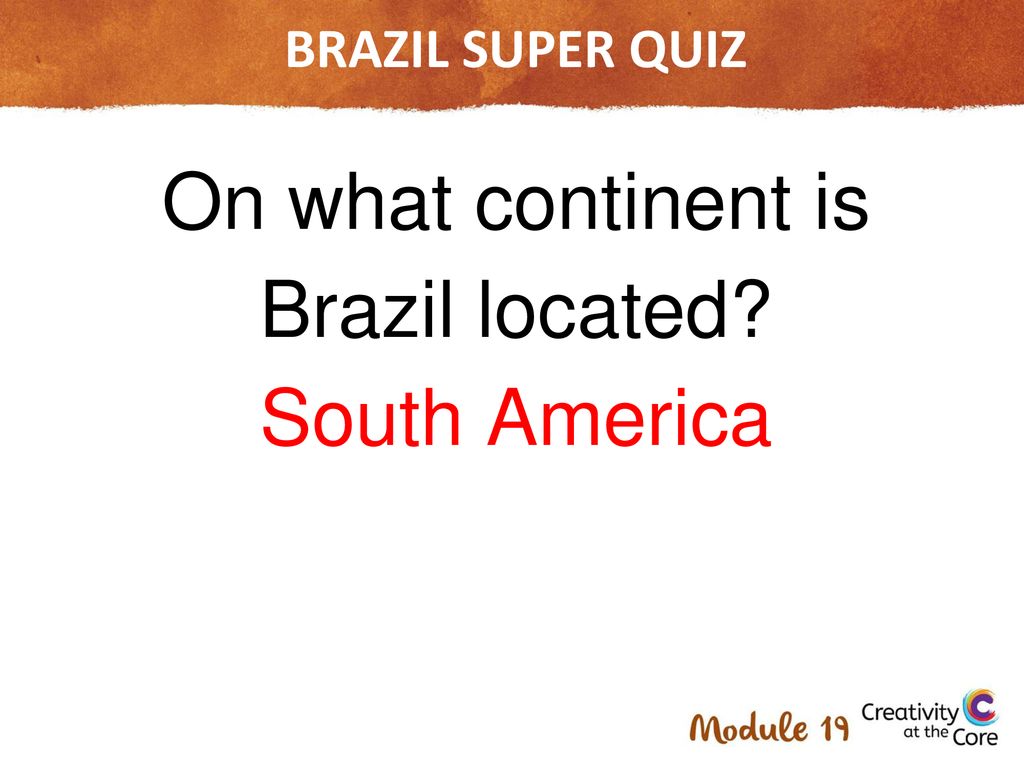The image features a quiz-themed design with a rugged, torn piece of brown paper at the top. Centered on this paper is the text "Brazil Super Quiz" displayed in white. Below this, on a white background, a question is presented in black text: "On what continent is Brazil located?" The correct answer, "South America," is displayed underneath in bold red text. 

In the bottom right corner, "Module Number 19" is elegantly written in cursive red font, followed by the phrase "Creativity at the Core" in standard black text. Above the word "Core" is a large, stylized letter "C" with a colorful outline: dark blue on the inside, transitioning to an orangish-yellow, then red, and finally edged with a baby blue.